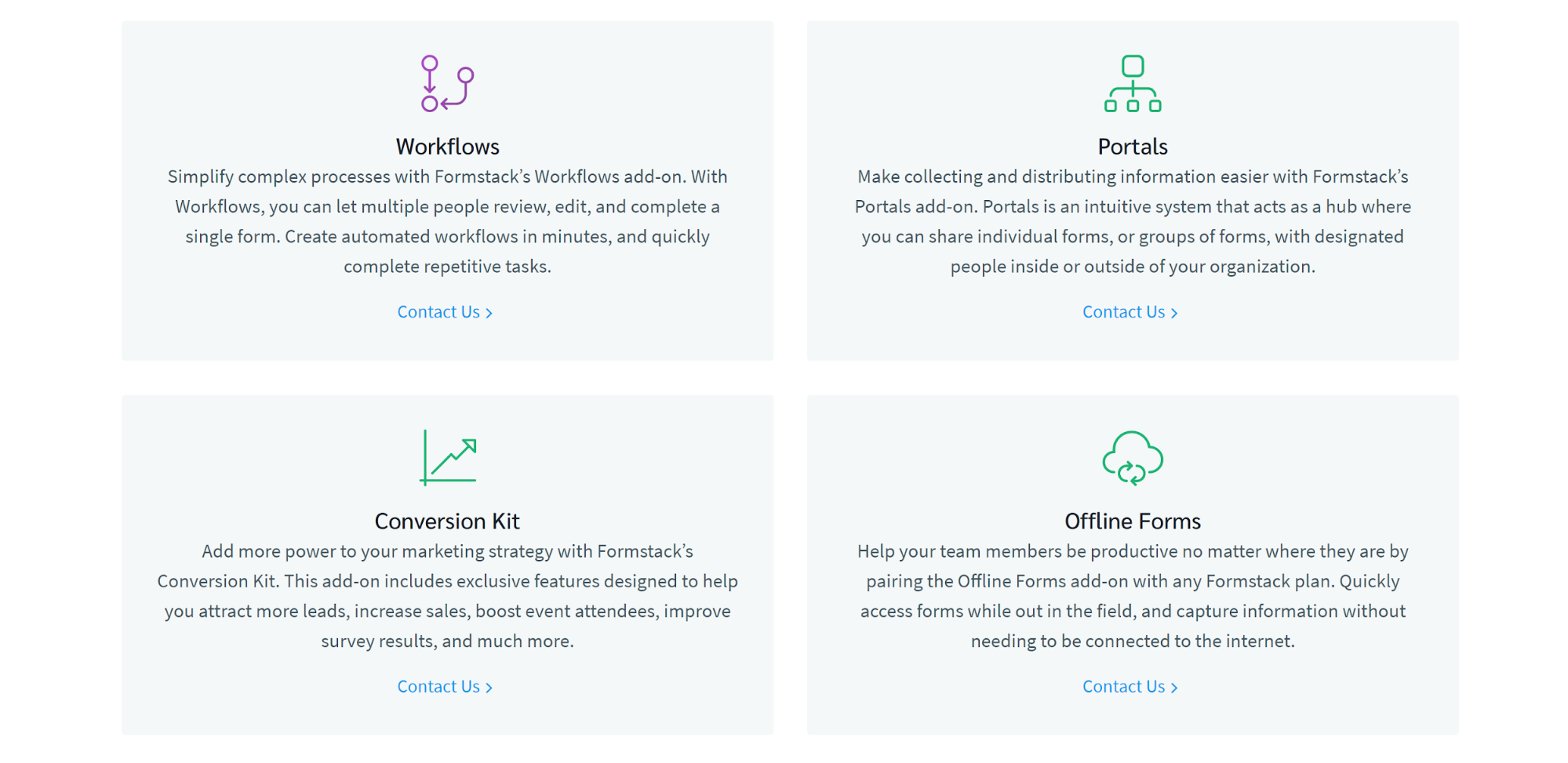**Image Description:**

The image is divided into four quadrants, each separated by white lines against a gray background. Each quadrant presents a feature of Formstack with a short description and a "Contact Us" link in blue.

1. **Workflows:**
   - **Graphic:** A purple icon with arrows and circles.
   - **Description:** "Simplify complex processes with Formstack's workflows add-on. With workflows, you can let multiple people review, edit, and complete a single form, create automatic workflows in minutes, and quickly complete repetitive tasks."
   - **Link:** "Contact Us" in blue.

2. **Portals:**
   - **Graphic:** None specified.
   - **Description:** "Make collecting and distributing information easier with Formstack's portals add-on. Portals is an intuitive system that acts as a hub where you can share individual forms or groups of forms with designated people inside or outside of your organization."
   - **Link:** "Contact Us" in blue.

3. **Conversion Kit:**
   - **Graphic:** None specified.
   - **Description:** "Add more power to your marketing strategy with Formstack's conversion kit. This add-on includes exclusive features designed to help you attract more leads, increase sales, boost event attendees, improve survey results, and much more."
   - **Link:** "Contact Us" in blue.

4. **Offline Forms:**
   - **Graphic:** None specified.
   - **Description:** "Help your team members be productive no matter where they are by pairing the offline forms add-on with any Formstack plan. Quickly access forms while out in the field and capture information without needing to be connected to the internet."
   - **Link:** "Contact Us" in blue.